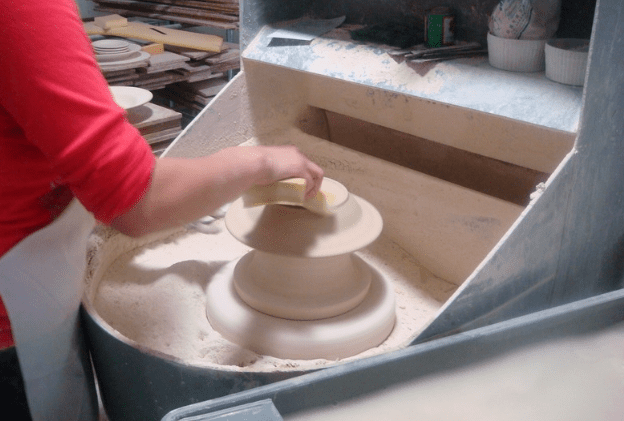A potter, dressed in a rolled-up red shirt and possibly blue jeans, is intently working on a large, electric potter's wheel. The artisan, potentially a woman, uses her right hand to smooth the bottom of a shallow bowl or plate, employing what might be a small block of wood. Surrounding her workspace, various tools for engraving and patterning sit neatly, hinting at the detailed craftsmanship involved in the process. Behind her, several completed ceramic plates are displayed, suggesting the piece she’s currently working on could align with these finished works. She is wearing a white apron, indicative of her dedication to this meticulous art form. The potter's wheel itself is notable for its size and complexity, signifying a professional setup distinct from smaller, pedal-operated versions.